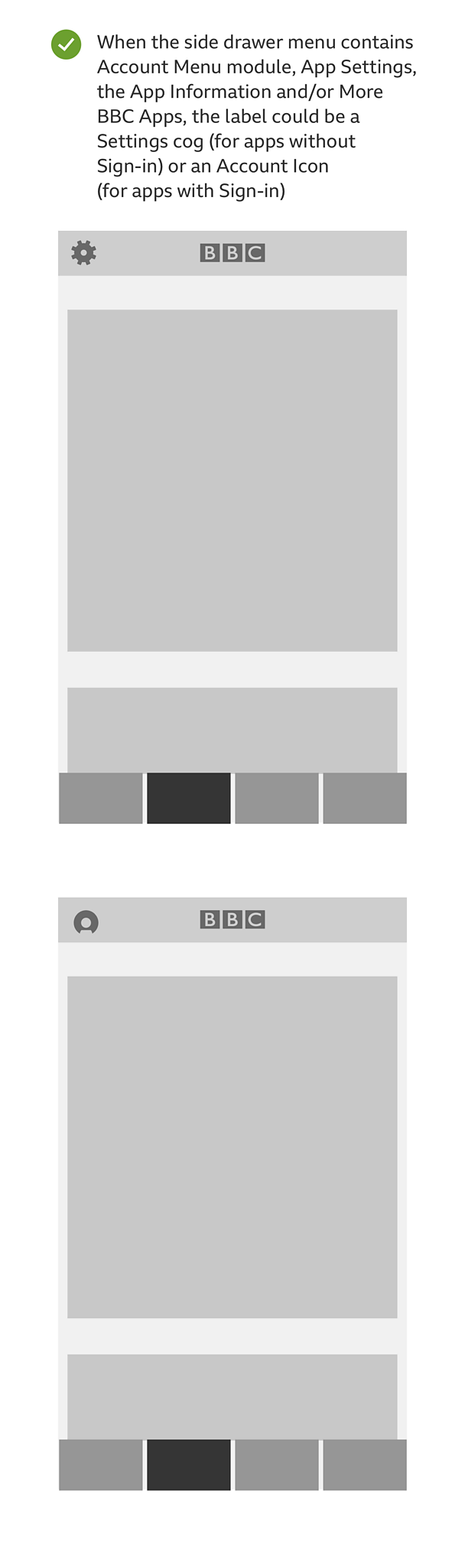This is a detailed caption of a cell phone screenshot displaying information related to BBC accounts. At the top of the screenshot, there is a green circle with a white checkmark inside it. Adjacent to the green circle is a concise tip in small black font explaining how to access various settings and menus within the BBC app. It reads: "When the side drawer menu contains account menu module app settings, app information, and more BBC apps, the label could either be a settings cog for apps without sign-in or an account icon for apps with sign-in." Below this tip, there are two small, empty gray boxes. Each gray box has a label at the top; the first one has a gear icon, and the second one has an avatar icon. The letters "BBC" are present within each gray box, which indicates different sections. However, these sections are devoid of any content. This could imply that the user is in the initial stages of the sign-in process or exploring navigation options within the BBC app.